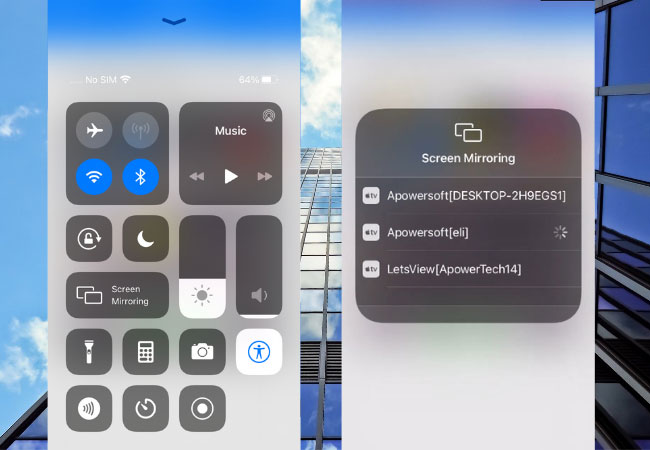This landscape-oriented image juxtaposes two mobile phone screenshots against a striking backdrop of a skyscraper viewed from below, soaring into a sky dotted with clouds. The skyscraper's reflective glass surface captures and mirrors the vibrant blue sky, adding an element of cohesion to the composition.

The left screenshot displays a rich, gradient background transitioning from light grey to dark blue at the top, where a status bar shows "No SIM" and a full Wi-Fi signal on the left, along with a 64% battery icon on the right. Below the status bar, a series of dark grey boxes offer several phone settings. The first box on the left contains four circles with white symbols: an airplane, a signal, Wi-Fi, and Bluetooth. Adjacent to it is a box marked "Music," featuring playback controls.

Further down, a small box with a white padlock icon encircled by an arrow appears, followed by another box displaying a moon symbol. Below these are options for "Screen Mirroring," identified by two overlaid screen icons, and four additional square icons: a flashlight, calculator, sound, and clock. To the right, three more icons are found—one for the camera, a white circle within a larger grey circle, and brightness and volume controls depicted by rectangles, with the brightness bar having a sun symbol and the volume bar nearly empty. Lastly, a white box with a blue stickman inside a circle is located at the bottom.

The right-hand screenshot features the same light grey to blue gradient background. Dominating the center is a large grey square with white text that reads "Screen Mirroring," accompanied by two overlaid box icons. Below, three Apple TV options are listed against a darker background with white text: "APOWERSOFT," "DESKTOP 2H9EGS1," and "APOWERSOFT ELI," the latter with a loading symbol. An additional option, "APOWERTECH 1-4," appears at the bottom. Each listing is prefaced by a white Apple TV logo.

Together, these elements craft a visually rich and detailed image, balancing the functional specificity of smartphone settings with the dynamic elegance of architectural photography.